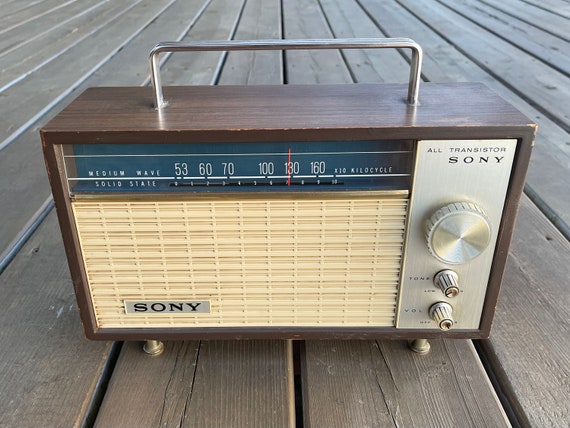The image showcases a vintage Sony radio, exuding an old-world charm. The radio is placed on a weathered wooden deck, with the dull brown planks displaying a pronounced wood grain and noticeable cracks, adding to the rustic ambiance. 

The radio, encased in a rectangular brown wooden frame, is elevated slightly by petite metal feet. A sleek silver handle arches gracefully from the top of the case. The front of the radio features a cream-colored waffle pattern, with a metal plate embossed with the brand name "Sony" prominently positioned. 

Adjacent to this, on the right side, a polished silver panel houses three silver dials – one larger and two smaller ones below it. Above these dials, engraved in the panel, it reads "All Transistor Sony". The top of the panel is adorned with a black strip, which includes a visible dial indicator showing the current frequency to which the radio is tuned. The overall composition of the radio and its surrounding elements creates a picturesque snapshot of nostalgic technology.